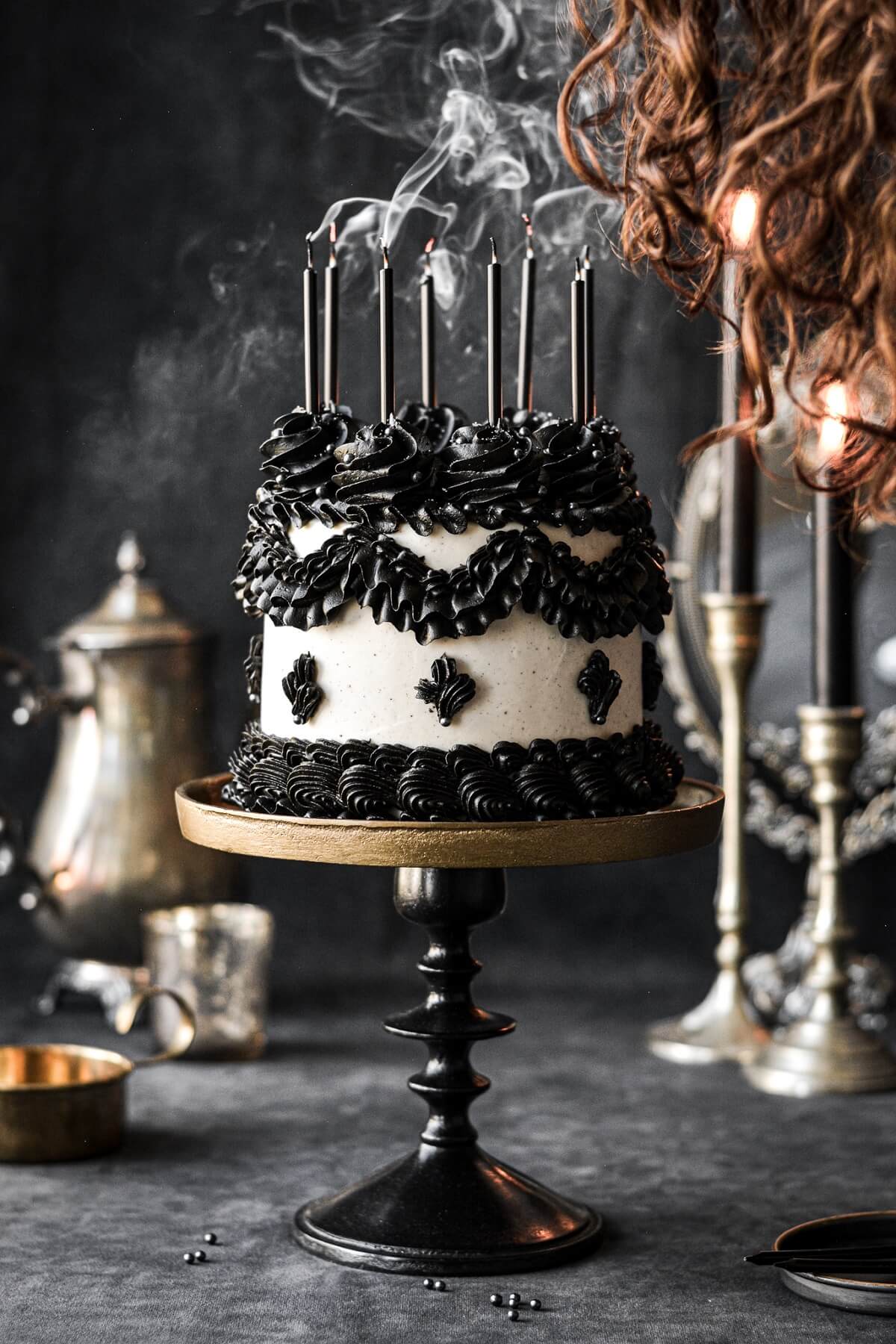The image portrays a striking three-layer cake adorned with contrasting black and white frosting. The cake's exterior features a base layer of white frosting, detailed with black designs spaced every few inches. A black scalloped frosting layer encircles the bottom, with another sweeping upward and downward along the middle. Atop the cake, an elegant arrangement of thick black rosette-like flowers supports several black birthday candles, some still faintly aflame while others emit curling wisps of smoke, suggesting they were just blown out.

This intricate confection is displayed on a tall, elegant cake stand, featuring a brownish-gold plate and a black wooden pedestal, and set against a dramatic black tablecloth. To the right of the cake, there are lit votive candles in silver candlesticks, and a silver platter leaning against an unseen support. Also visible is a glimpse of someone's red wavy hair hanging over the table.

In the background, to the left of the cake, stands a silver coffee or teapot accompanied by a matching glass and a copper-colored ashtray-like object. Additional details include some beads scattered on the tablecloth, a small tray with a black pen, and a muted background that enhances the cake’s elaborate presentation.